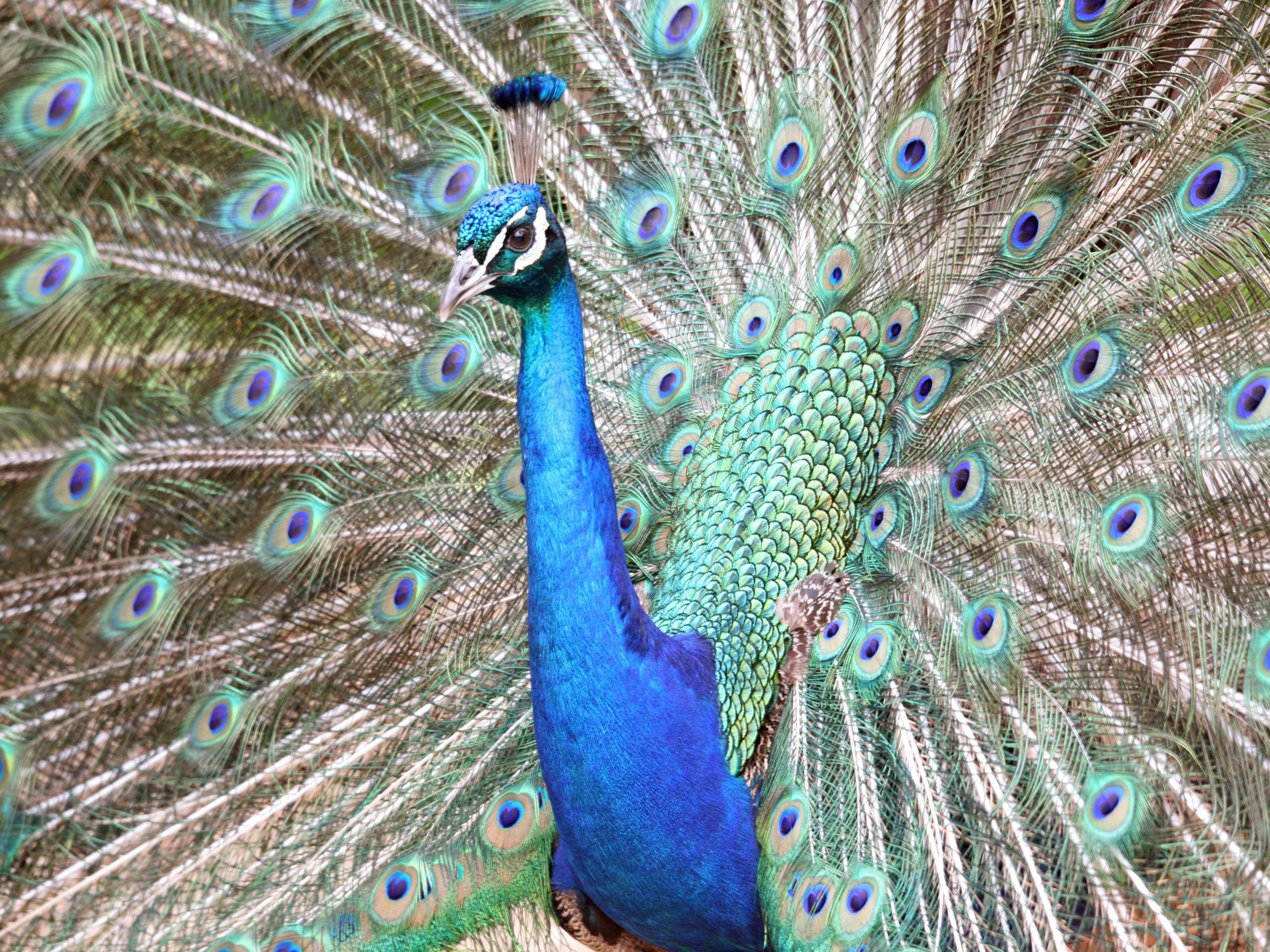A striking image of a male peacock dominates the scene, showcasing its vibrant and elaborate plumage. The peacock is centrally positioned, with its head turned slightly to the left, allowing a glimpse of one black eye and its pointed, brown beak. Its head is adorned with small blue feathers extending upwards, and two distinctive white lines frame its eyes. The peacock's neck is a vivid blue, seamlessly transitioning into a solid patch of green feathers on its back. From this patch, an impressive fan of decorative feathers radiates outwards, nearly filling the frame and extending to the edges.

These feathers are intricately detailed, with a cascade of colors—blues, greens, and browns—culminating in numerous eye-catching circles. Each circle features a teal outer ring, followed by a brown band, and a blue center with hints of black. The feathers create a mesmerizing pattern that contrasts subtly with the barely visible white background peeking through. The overall composition highlights the peacock's natural splendor and the symmetrical beauty of its fanned-out tail, reinforcing why this bird is a symbol of elegance and pride.